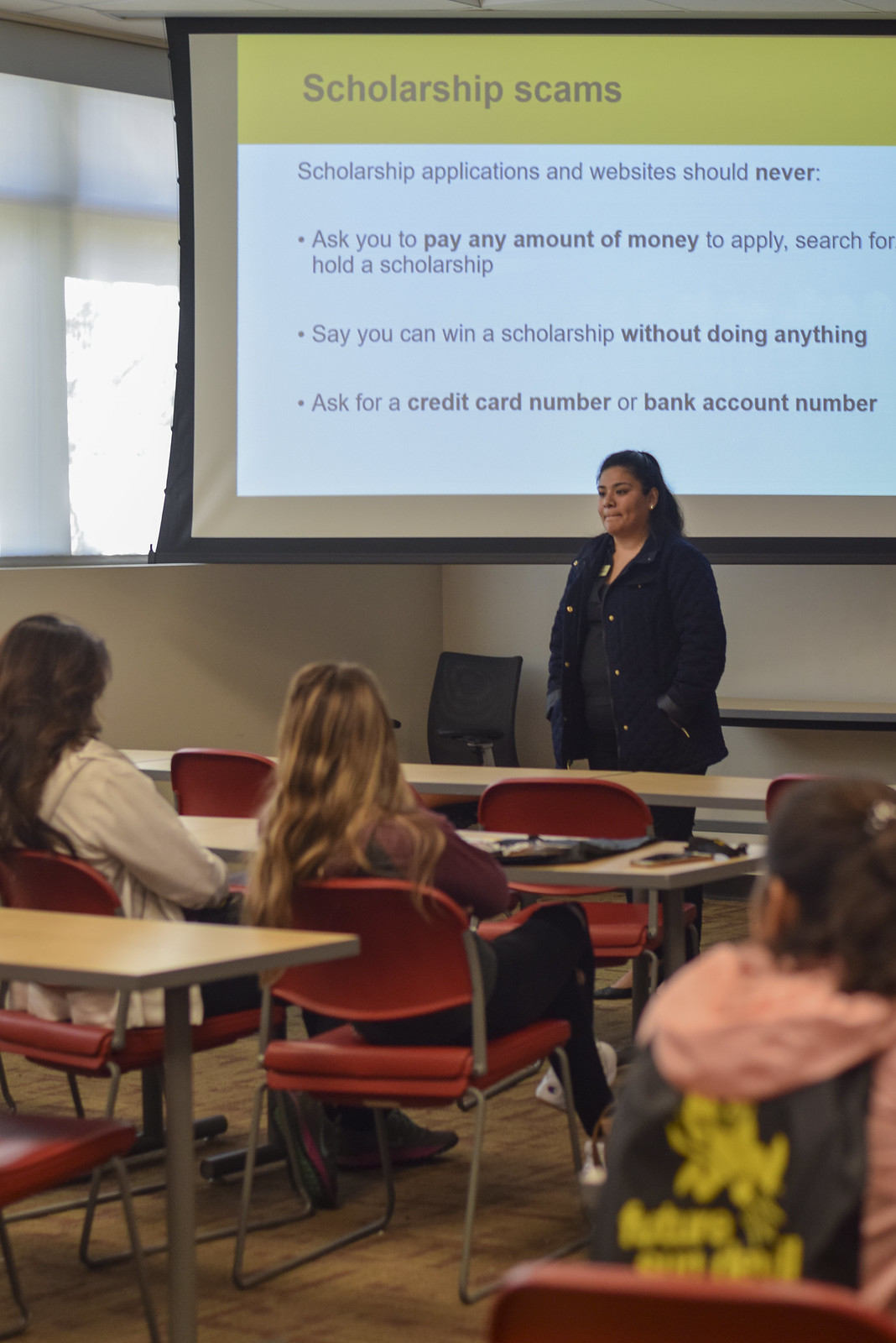This vertically aligned rectangular photograph captures a woman with shoulder-length black hair pulled back, dressed in a black jacket over a dark gray shirt, standing at the front of a classroom. In the background, a screen displays the title "Scholarship Scams" in gray text against an olive green background, with three warning bullet points underneath on a white backdrop. The text reads: "ask you to pay any amount of money to apply, search for, or hold a scholarship," "say you can win a scholarship without doing anything," and "ask for a credit card number or a bank account number." In the classroom, the walls are white and the chairs are red. Three high-school-aged students, visible from the back, are seated at desks, with one on the far right wearing a pink hooded jacket with black and yellow writing, though she appears slightly blurred. The image clearly conveys the lesson focus, highlighting the warning signs of fraudulent scholarship offers as part of the educational session.